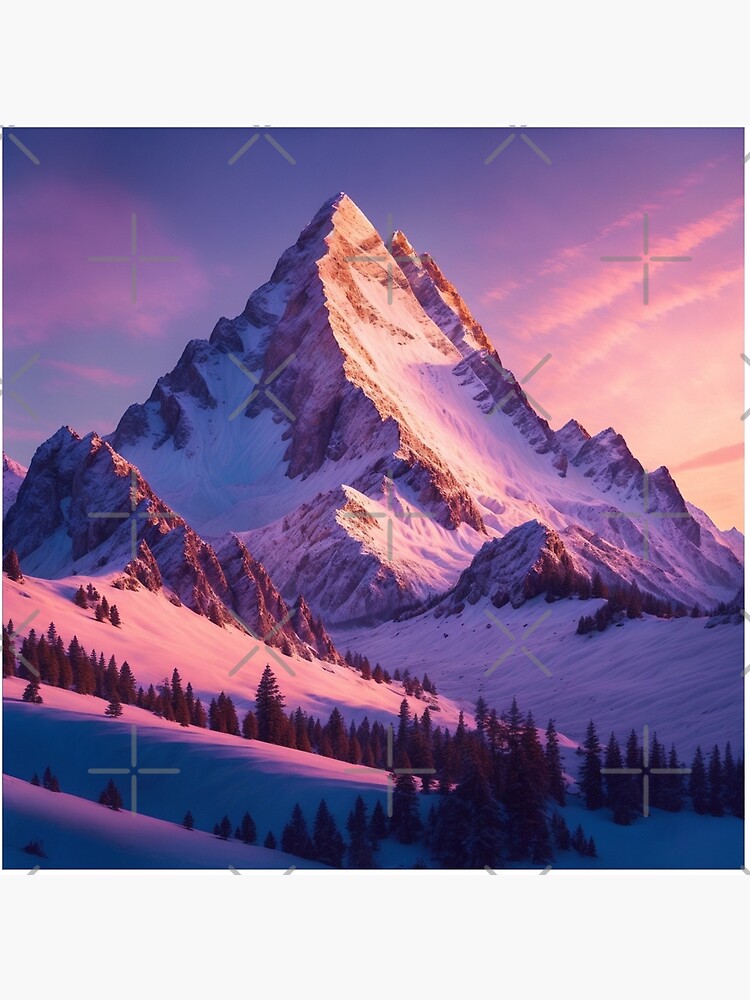The image depicts a majestic, pyramid-shaped mountain that has likely been sculpted by glaciers, featuring steep and jagged snow-covered sides. The mountain's peak narrows into a point, while its broad base supports a picturesque landscape of valleys and rocky outcroppings. Evergreen pine trees are scattered at the base, where lower altitudes allow for their growth. The mountain is reminiscent of the iconic peak from the Paramount logo, standing tall and almost inaccessible, with city officials having restricted access due to its extreme elevation. Interestingly, the surface of the image has small X marks, possibly indicating civil engineering elevation measurements. The lighting in the scene is striking, with the right side of the mountain bathed in pinkish sunlight, creating a beautiful contrast with the shaded, bluish-purple hues on the left. The sky above adds to the ethereal quality of the image, showing gradations from a clear blue on the left to pink and white towards the right, interspersed with light clouds tinged with pink and white. The overall effect is a stunning depiction of a towering, natural pyramid amidst a tranquil, snowy landscape.